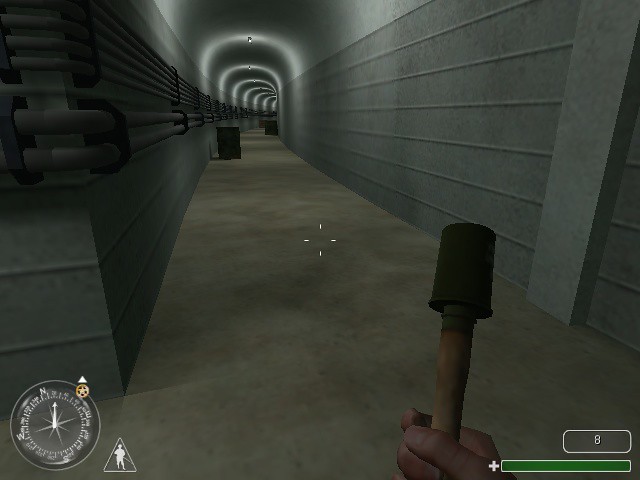This screenshot from a computer game showcases a first-person view of a character navigating a dark gray, stone corridor that slightly curves to the right at the end. The corridor features an arched ceiling with vertical and horizontal lines. The ceiling's color gradient transitions from light gray to darker shades towards the curved end. The pathway and ceiling are illuminated at regular intervals by lights installed overhead. Notably, gray pipes run along the entire length of the left-hand wall.

In the bottom right corner of the screen, the character's hand is visible, holding an unlit torch-like object with a wooden handle and a black, cup-shaped top, resembling the flammable part of a torch. A Heads-Up Display (HUD) is present, featuring a white-bordered rectangle displaying the number 8, a longer green rectangle likely representing health points (HP) with a white plus sign to its left. A white circular compass occupies the bottom left corner, with directions marked and a white arrow pointing slightly to the right of north. Scattered across the corridor floor are black, cylindrical objects at regular intervals. The overall atmosphere suggests an underground tunnel or bunker with a detailed and immersive first-person perspective.